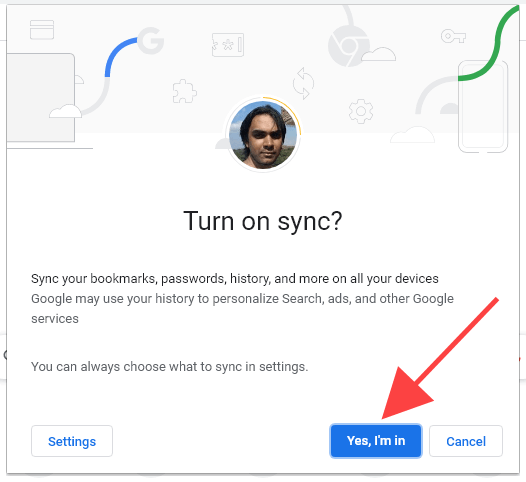The image displays a screen prompting the user to "Turn on sync?" for Google services. At the center of the screen, a face possibly belonging to a Middle Eastern or Indian man is visible, likely indicating his account. Above his head, various icons are displayed, including a grayed-out Chrome logo, a Google 'G' logo, a phone, a key, a laptop, and a cloud, suggesting services and devices that can be synced.

Underneath his image, the text reads: "Turn on sync?" with a description explaining, "Sync your bookmarks, passwords, history, and more on all your devices. Google may use your history to personalize search ads and other Google services. You can always choose what to sync in settings."

At the bottom left corner, a "Settings" button allows the user to customize sync options. On the right, a blue button labeled "Yes, I'm in" is prominently highlighted with a red arrow pointing towards it, encouraging the user to click it. Adjacent to this is a "Cancel" button for opting out.

The screen features a simple white background with black text, creating a clean and straightforward interface.